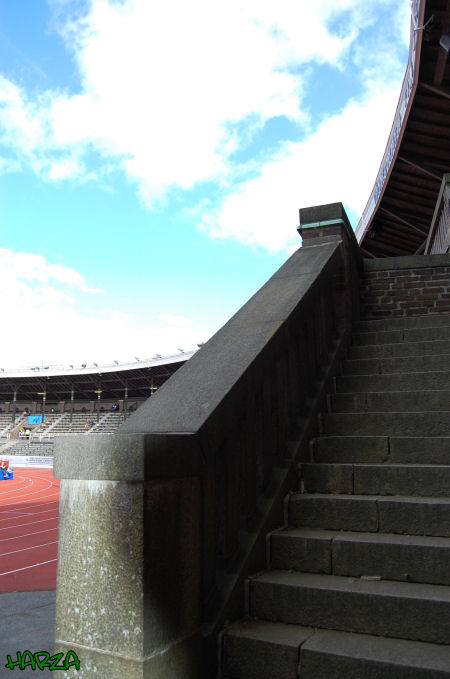This photograph captures a detailed partial view of a track stadium, likely at a school. Dominating the right side of the image is a broad cement stairwell, featuring a substantial cement handrail, quite different from typical thin metal rails. The stairwell appears to lead up towards the stadium seating. In the background, you can glimpse the amphitheater-style seating that circles the track, indicating a circular stadium layout.

To the left of the stairwell and beneath the seating, a section of the running track is visible. This track is characterized by its brownish-red surface adorned with white lines, forming the lanes. The vibrant sky overhead features a mix of bright blue and turquoise hues, punctuated by fluffy white clouds.

The lower-left corner of the image includes green text, "Harza," which likely credits the photographer. The scene is tranquil with no people or motion, featuring just the static architectural elements against a lively sky.